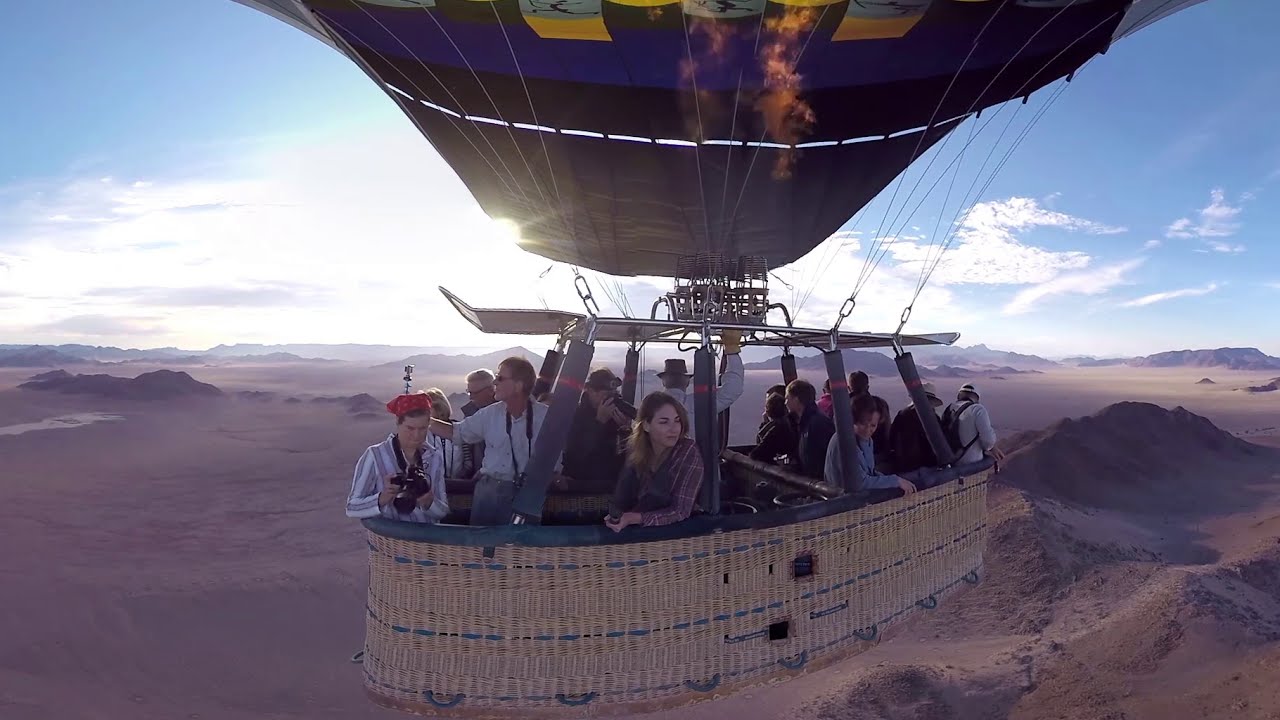This outdoor photograph captures the intriguing sight of a hot air balloon in flight during the daytime, set against a clear blue sky dotted with clouds. We observe the gondola, or basket, of the balloon from an aerial perspective. The basket is crafted out of wicker with a light brown hue, accented by blue stitching that runs throughout its long, oval shape with slightly pointed ends. It features a mix of blue tethers for securing to the ground and metal posts topped with dark blue cushions edged with red rings, ensuring passenger safety and comfort.

Inside the basket, two groups of tourists are arranged, flanking the central area reserved for the balloon operator. Seven people each occupy the front and back sections, while the operator, donning a long-sleeved white shirt, a hat, and a yellow glove on his right hand, manages the heating mechanism that propels flames into the balloon above. These flames keep the deep blue balloon, which is adorned with yellow writing and squares, aloft.

One notable detail is a woman within the basket holding a camera, capturing the moment from her unique vantage point. Beneath them, the terrain stretches out in a possibly desert-like landscape, marked by barren, brown flatlands and rocky, undulating hills, devoid of any greenery. The entire scene conveys a sense of serene adventure amid the vast, untouched expanse below.